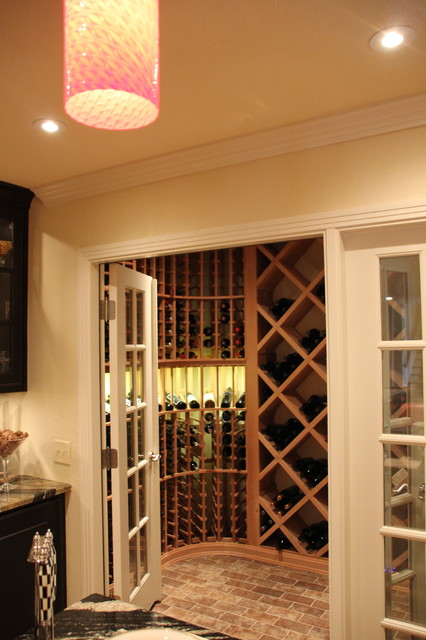The image depicts a luxurious walk-in wine cellar situated adjacent to a kitchen-like area. The wine storage room is accessed through white-paneled glass doors that are flanked by wooden frames. Inside, the light beige walls and ceiling create a soft ambiance, accentuated by recessed lighting and a prominent pink lamp dangling from the ceiling. The floor of the wine room is lined with pale reddish-brown brick tiles. On the left side of the room, vertical shelves neatly stack wine bottles, while the right side houses shelves with a diamond-shaped design, allowing the bottles to nestle together. Outside the wine cellar, there is a marble countertop, partially visible, adorned with a cylindrical red and yellow lamp. Below, a black cabinet with glass doors is noticeable against the tan walls. The countertop also includes a container filled with brown items and a couple of light switches, completing the scene of opulent design and functionality.